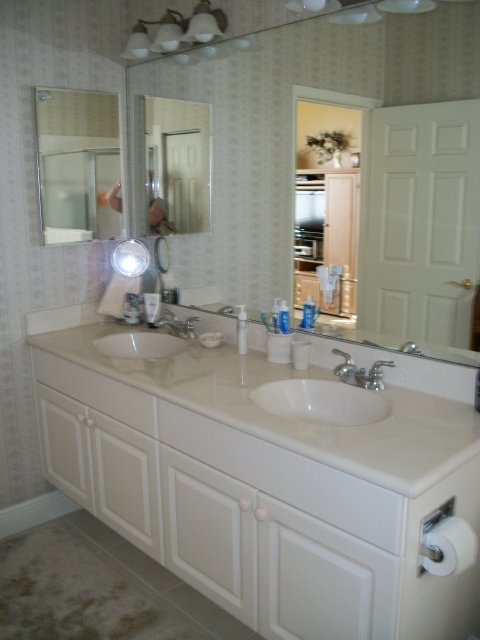The photograph captures a pristine home bathroom interior, focusing on a rectangular sink counter that dominates the central portion of the image. This long, white countertop features two embedded sink basins, each adorned with stainless-steel faucets equipped with separate hot and cold water taps. Above the counter stretches an expansive mirror, reflecting the scene behind the photographer - a cozy living room furnished with a wooden entertainment console and a TV, visible through a white door frame. The bathroom door, also white with a brass handle, stands open, providing a glimpse into the adjoining room. In the bottom right corner of the image, a stainless-steel toilet paper holder is conspicuously mounted to the side of the bathroom cabinetry, holding a roll of toilet paper. The overall composition is rectangular, with the longer sides on the left and right, offering a comprehensive view of this elegant and functional bathroom space.